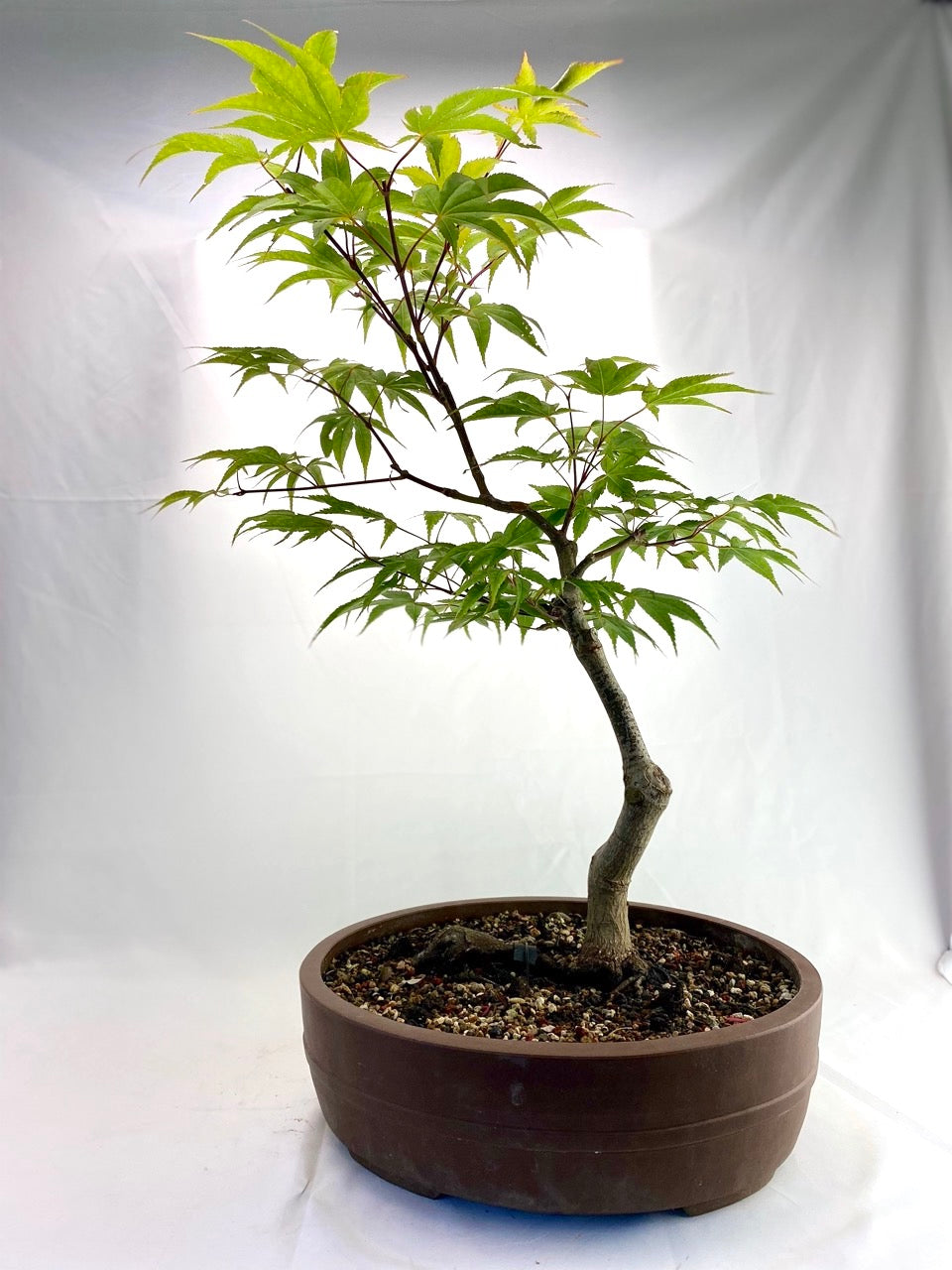This color photograph captures a well-rooted bonsai tree, possibly a maple, planted in a not-very-deep, circular brown clay pot filled with regular soil speckled with small white particles, potentially fertilizer. The tree, about 12 to 18 inches tall, features a thick stem that bifurcates into thinner branches all adorned with green leaves. The setting includes a white sheet draped behind and beneath the tree, functioning as a wrinkled homemade lightbox backdrop to accentuate the bonsai’s detailed form and heighten its visual contrast.